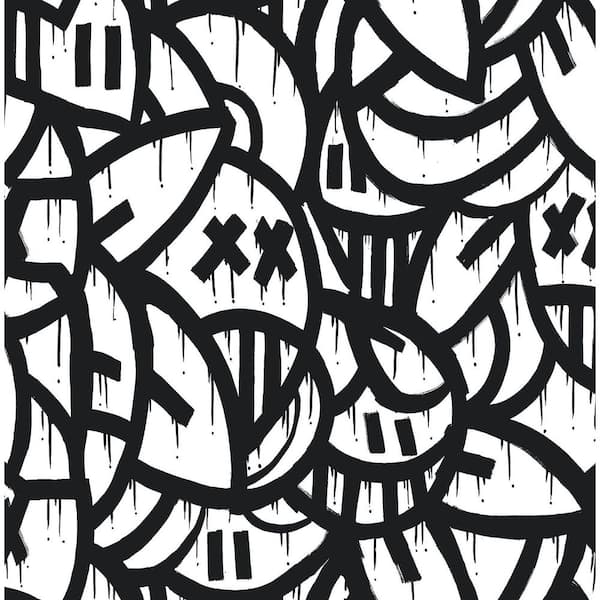The image features an intricate black and white art piece set against what appears to be a white background or canvas, possibly framed with wood. The artwork consists of a chaotic yet deliberate arrangement of various shapes and lines. Dominating the scene are thick black lines that intersect and overlap to create partial figures, circles, cones, and other abstract forms. Among these shapes are an array of smaller black lines reminiscent of exclamation points, as well as numerous X's and O's distributed throughout the piece.

More detailed observations include two thick vertical black lines located at the top left, resembling a rotated equal sign, with similar lines appearing intermittently in other sections. There are pairs of large black X's, notably in the middle left and the right side of the image slightly above center, one extending beyond the frame. The composition evokes a sense of spontaneous creativity, with paint seemingly applied in unrestrained, dripping strokes that encompass a variety of forms such as half circles and ambiguous shapes that may suggest ears or smiles with teeth. Despite the apparent randomness, no single line bisects a circular shape completely, and no entirely vertical lines dominate the scene, contributing to its profound complexity and abstract nature.